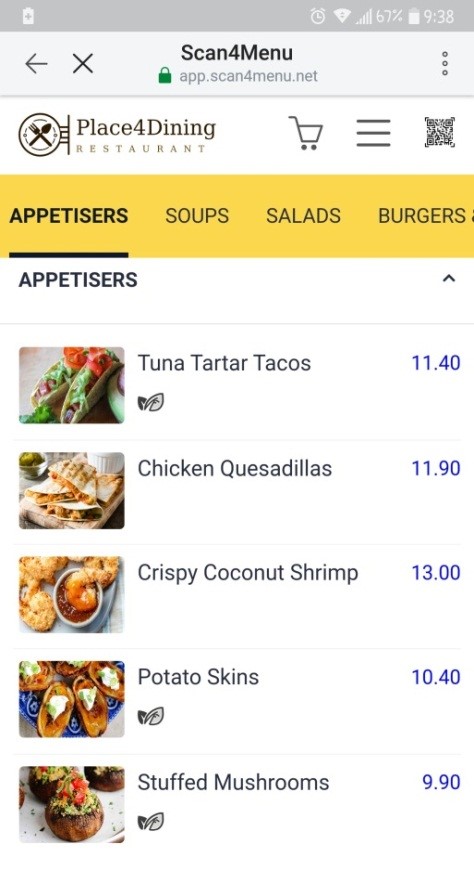A smartphone screen displays a dining website, specifically the “app.scanformenu.net” for "Place for Dining Restaurant", featuring various menu categories and items. The device status bar at the top shows a partially charged battery at 67%, actively charging, with a Wi-Fi connection and an alarm set at 9:38. The time is indeterminate between AM or PM. Below the status bar, a light gray navigation bar includes a green padlock icon beside the URL app.scanformenu.net, a back arrow, an “X” for closing, and a three-dot menu icon. Beneath this, the website header features the restaurant’s name, represented as "Place 4 Dining Restaurant", accompanied by an icon of a plate with a fork and spoon crossed over it. Also present are icons for a shopping cart, and a menu represented by three horizontal lines, along with a QR code for quick access. The menu section highlights categories: Appetizers, Soups, Salads, and Burgers, with "Appetizers" prominently underlined. Below the appetizers section, dishes such as Tuna Tartar Tacos, Chicken Quesadillas, Creamy Coconut Shrimp, Potato Skins, and Stuffed Mushrooms are listed, each with accompanying images.